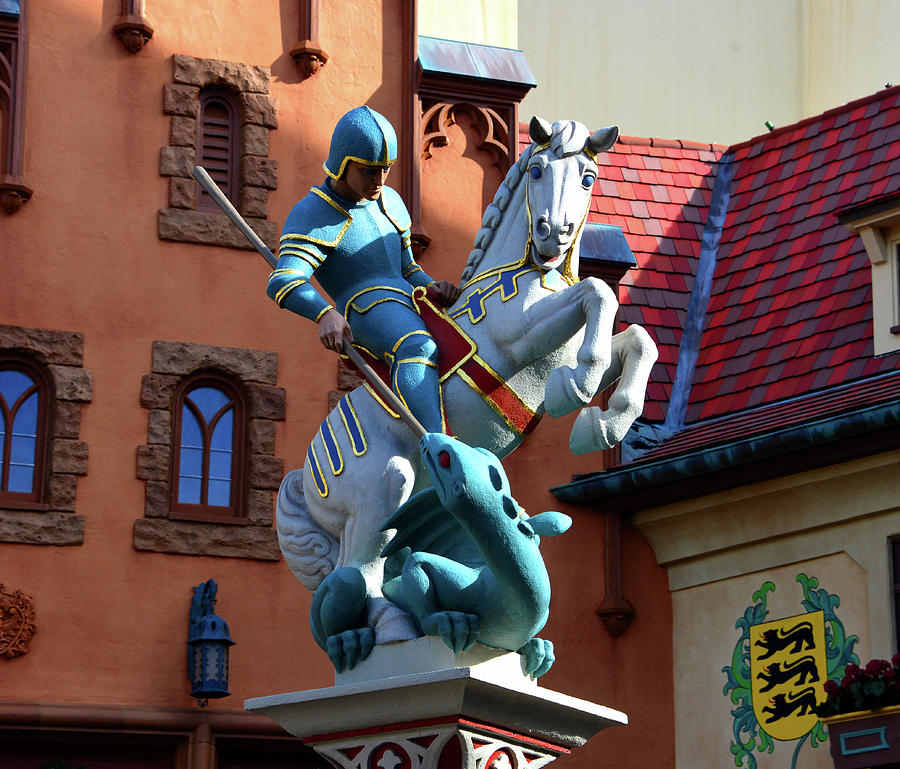In this vividly detailed image, we see a striking statue that appears to be a combination of a painted sculpture and possibly a digital render. It features a dynamic scene of a knight on a rearing off-white horse, battling a serpentine dragon in what seems to be a medieval town square. The horse, detailed with bright blue eyes, is adorned with a red saddle trimmed in gold and a blue harness with gold accents. The knight, clad in striking blue and gold armor, wears a matching helmet as he thrusts a spear down at the dark blue, scaly dragon below.

The statue is mounted on a white pedestal with red trim, adding to its grandiose presence in the square. The backdrop is a vivid cityscape with buildings in varied bright colors. To the right, there is a tan building featuring a yellow coat of arms with three large black cats, adding a heraldic touch. Another building is notable for its vibrant orange color and blue-tinted windows, as well as a blue lantern mounted on its wall. Roofs in the background add to the colorful scene, with tiles in a striking mix of purple, pink, and red. This dynamic tableau, rich in color and detail, blends elements of reality and artistic fantasy, making it a captivating focal point in this medieval-like setting.